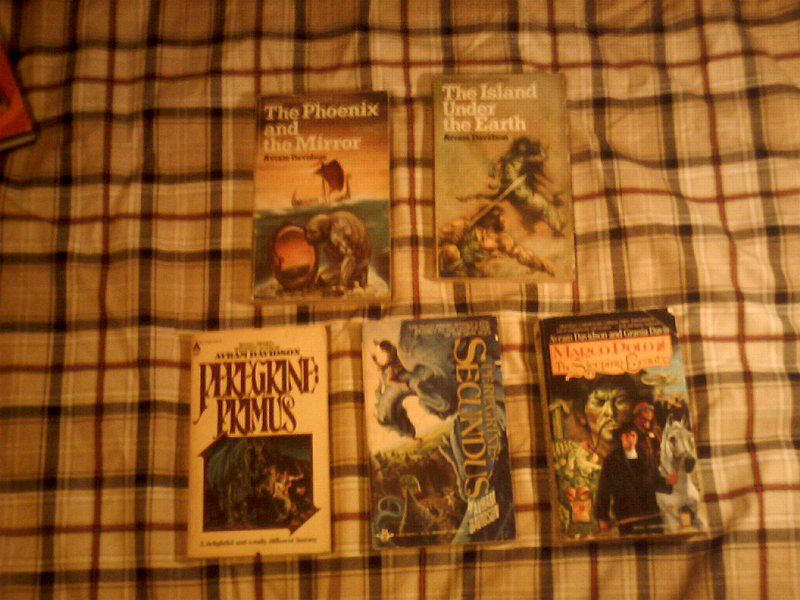This is a photograph taken from above, capturing the front covers of five small paperback books arranged on a cream-colored, plaid fabric featuring light brown, dark brown, and dark red checkered patterns. The books appear to be of the same genre and possibly by the same author, though the name is unclear due to the blurriness of the image.

At the top left, we see "The Phoenix and the Mirror" with a brown top portion above an image featuring a body of water and a gray character. Next to it, "The Island Under the Earth" displays a cover with two people fighting in front of a blend of white, blue, and green designs. Below these two, to the far left, is "Pengreen Primus," characterized by a white cover with dark purple text. In the middle is "Secundus," recognizable by its yellow text on a background of white mixed with blue and green accents, though specific images are unclear. The book to the right is difficult to read but includes images of a horse, a man in a black suit, and a green face.

A small corner of an additional book is visible in the upper left-hand corner of the photograph, though its title and details are indistinct. Overall, the image captures a literary collection on a cozy fabric backdrop.